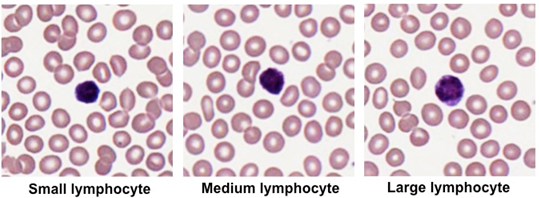The image displays three horizontal microscope photographs illustrating varying sizes of lymphocytes labeled as "small lymphocyte," "medium lymphocyte," and "large lymphocyte." Each photograph features a prominent purple central dot—indicative of the lymphocyte—surrounded by a cluster of smaller dots with pinkish borders and white centers. The first image with the label "small lymphocyte" shows a small, dark purple lymphocyte at its center. Moving to the "medium lymphocyte," the central dot remains darker purple, maintaining a similar dense arrangement of surrounding colored dots. The final image, labeled "large lymphocyte," displays a larger, less uniformly colored central spot exhibiting shades of violet, dark purple, and medium purple, along with fewer surrounding pinkish-white dots compared to the smaller lymphocytes. The labels beneath each image are presented in a bold, small basic font.